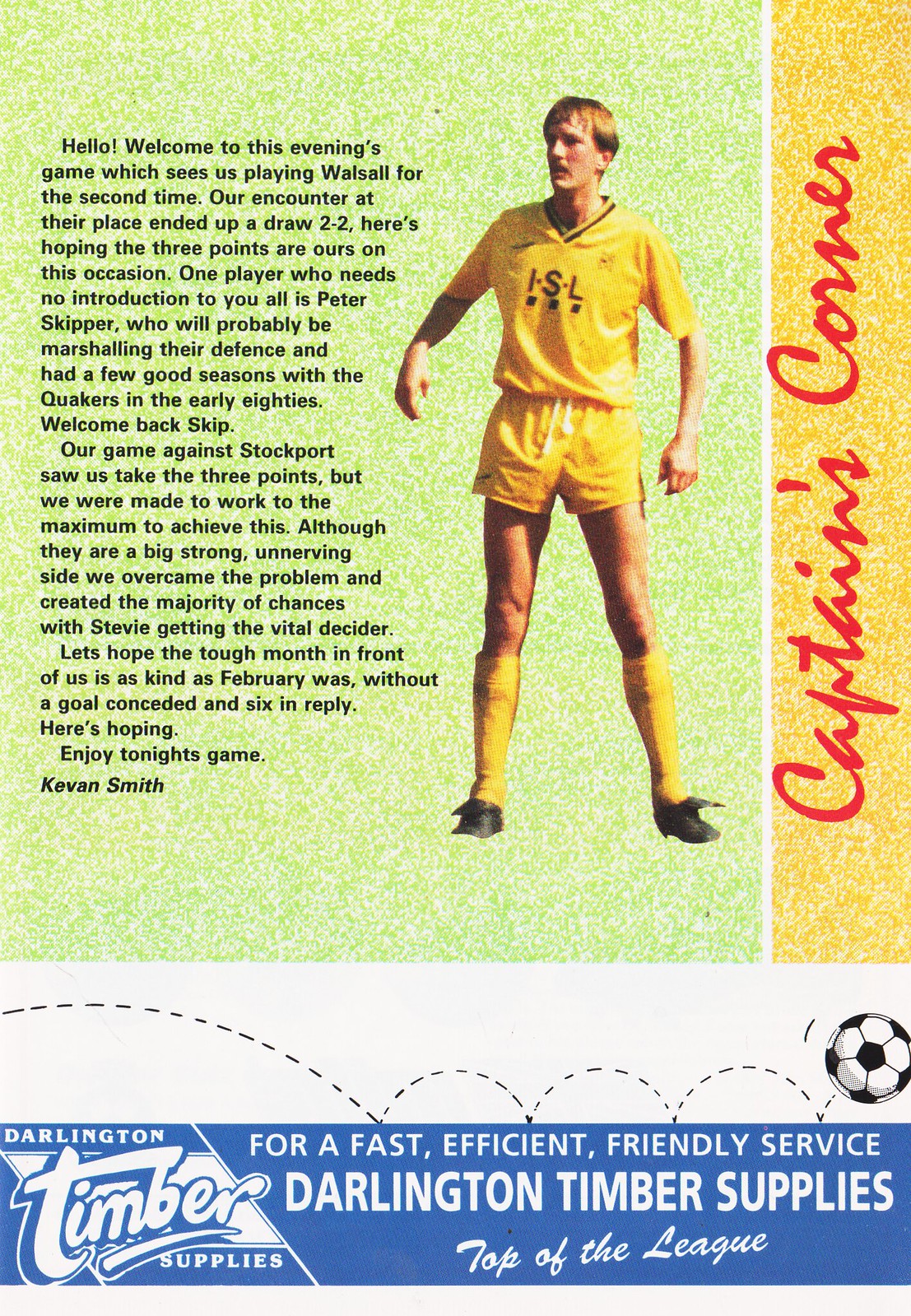The image appears to be a scanned portion of a vintage magazine or flyer, likely from a soccer event. Dominating the center is a photograph of a soccer player dressed in a yellow uniform—shirt, shorts, and socks—with black shoes. To the right of the image, in italic red cursive text, it reads "Christian Connor" vertically along a yellow bar. The left side of the image features detailed information about the evening's game, noting that they are playing against Walsall for the second time following a 2-2 draw in their previous encounter. This section also discusses the return of Peter Skipper, a formidable defender from the early 80s, and reflects on a recent victory against Stockport, highlighting the team's perseverance and goal-scoring prowess. The text, which seems to be a quote from Kevin Smith, ends with a hopeful message for securing three points tonight.

Below this narrative is a segment dedicated to promoting Darlington Timber Supplies. The advertisement includes their slogan, "For a fast, efficient, friendly service, Darlington Timber Supplies, top of the league," alongside a hand-drawn, bouncing soccer ball. To the far left, there appears to be another advertisement, written in red cursive text, though it is somewhat difficult to read. The background behind the advertisements consists of a green color with a white texture, adding a visually distinct element to the overall layout.